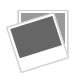This close-up image features a dark charcoal gray fabric with a prominent, textured surface. The fabric is densely detailed with a series of darker seams and lines that traverse the entirety of the material. The most noticeable features are two vertical seams that run parallel from the top to the bottom on the left-hand side. Additionally, there is a long, diagonal seam running from the top left corner to the bottom right corner. The fabric is punctuated by numerous small, rectangular stitching details, roughly about a centimeter long, which are unevenly spaced and form dashed lines. These lines run from the bottom to the top and from left to right, often overlapping and creating a complex, crisscrossing pattern across the fabric's surface. The texture is further defined by small, darker holes that enhance the overall intricate appearance of this deceptively simple fabric swatch.